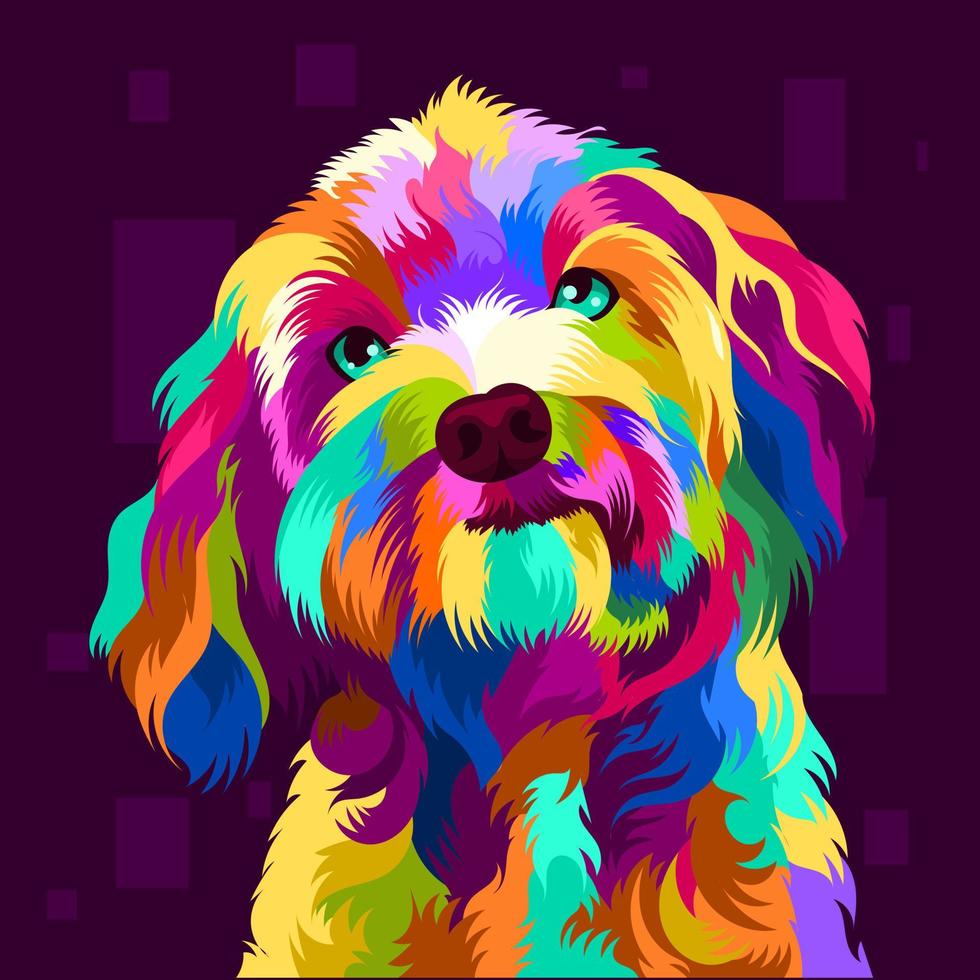This vibrant artwork depicts a fluffy, toy-like dog reminiscent of Benji from the Disney movie, with short hair around its face and long hair at its ears and neck. The dog's head is tilted slightly to the left, giving it a curious expression as it looks up with strikingly bright teal blue-green eyes featuring black pupils. The dog's fur is a dazzling array of rainbow colors: 

The top of its head has patches of yellow, transitioning to purple on the right and blue below. Around the nose, the fur turns from a pure white at the center to yellow, then green at the sides with purple and blue further out, framed by more yellow. The snout features a dark purple or brownish nose while the mouth area is adorned with both light and dark purple, transitioning to yellow and light blue below the nose.

Its neck area is a mix of darker blue and purple hues. The body shows a cascade of colors: starting with yellow on the left side, mingling with patches of green, light blue in the center, transitioning to orange and brown on the right with a final touch of purple and blue down the sides. The ears boast a mixture of purple, blue, and pink on the right, and blue with orange, brown, green, and pink on the left.

The background complements the colorful figure of the dog, painted in deep purples with lighter purple squares and rectangles scattered throughout, enhancing the overall vivacity of the artwork.